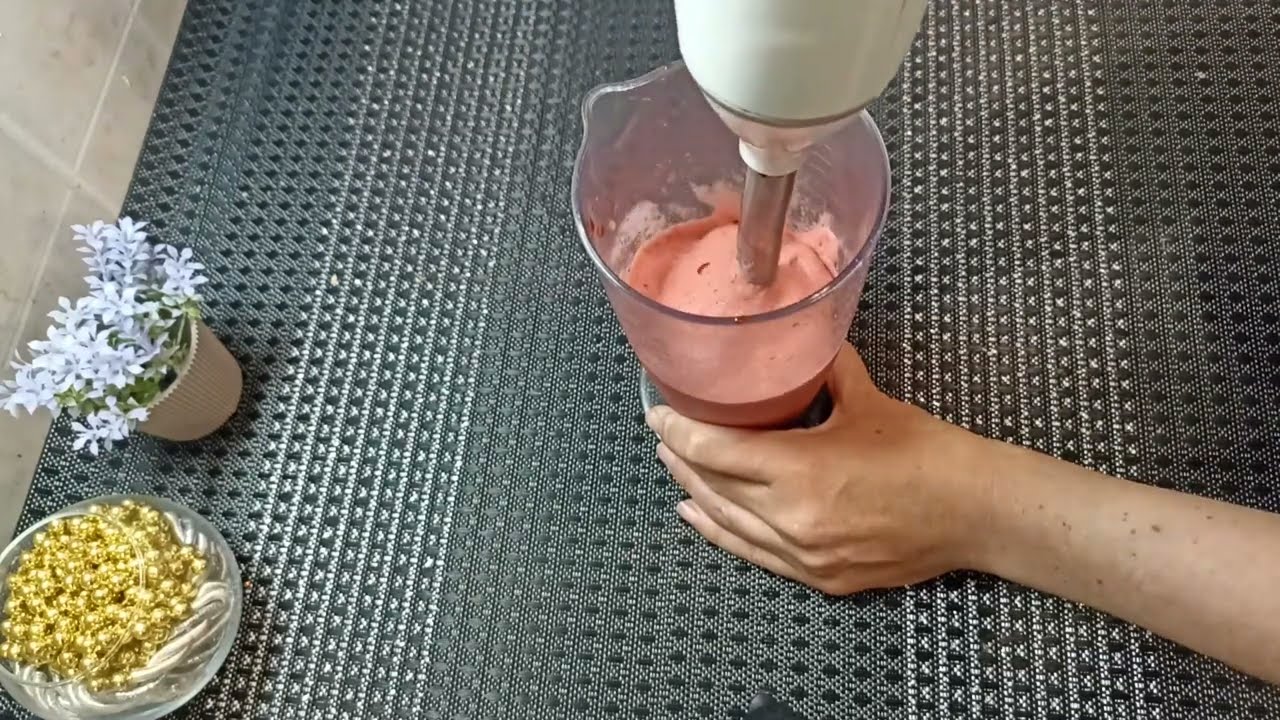In the photograph, a person is seen mixing a thick, pinkish-orange liquid, likely a smoothie, using a white and silver hand mixer. The concoction is in a large plastic pitcher, which the individual is holding with their left hand. The scene is set on a table or counter that is covered with a gray and white patterned mat. To the left of the pitcher, there is a small white flower pot with bluish-white faux flowers and a round glass bowl filled with shiny golden beads, reminiscent of festive decorations. The person's hand, appearing somewhat thin and without nail polish, is visible at the bottom of the image, firmly gripping the pitcher.